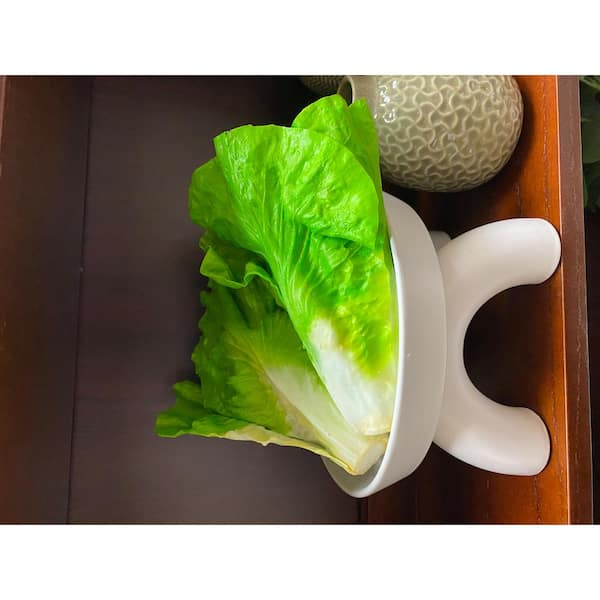The photograph, taken from an unusual sideways angle, features a horizontally oriented scene. At the center is a white ceramic bowl supported by two curved, macaroni-like legs acting as a base. Inside the bowl, two stalks of lettuce are visible; the green leaves contrast with the white stalks at the bottom. The nature of the lettuce—whether real or artificial—remains ambiguous. To the foreground, which would be the right in correct orientation, stands a small tan ceramic vase with a distinctive squiggly white pattern. This vase features a narrow opening at the top. The entire setup rests on a wooden table or shelf, which matches the wooden back wall, suggesting an encased, wooden space. The details of anything beneath the table or directly behind the vase are obscured.